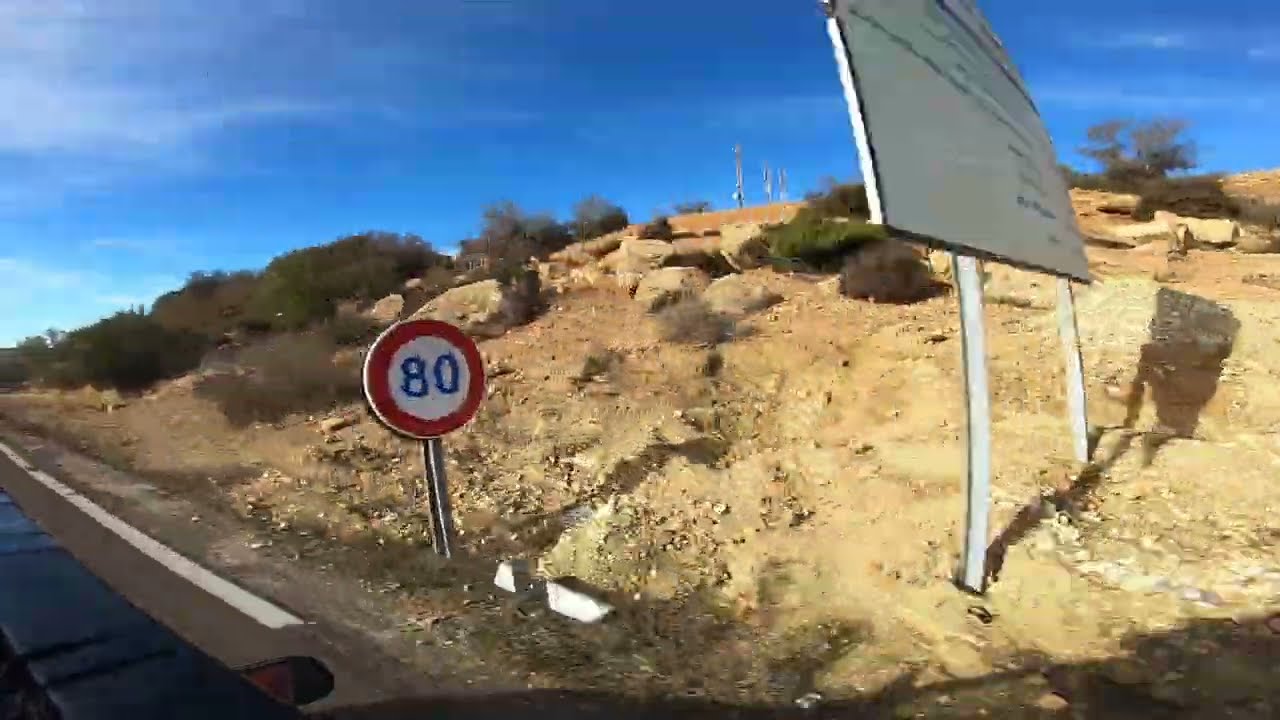The photograph, taken from a moving vehicle, captures the side of a road under a bright blue sky. In the bottom left corner, the car's side view mirror and a white road stripe are visible. The road is bordered by beige gravel and dotted with scrubby brush and green bushes. Prominently featured is a round road sign with a red border and a white center displaying '80' in blue text. Just before this sign, a larger white sign on two gray posts stands, though its text is unreadable. The image, slightly blurry from motion, shows a bright, daylight scene with clear rocky terrain and distant vegetation.